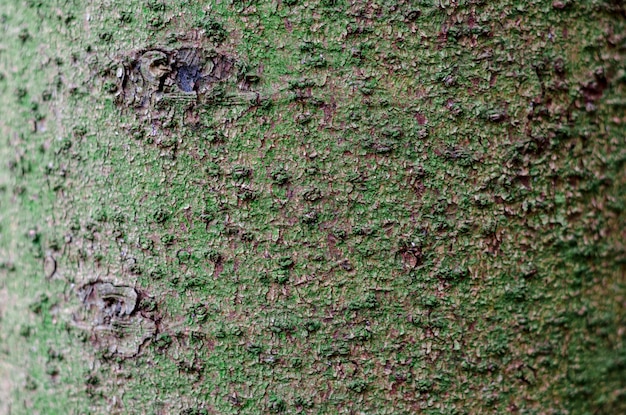This striking close-up image appears to capture the textured surface of a tree trunk, densely covered with green moss. The aerial-style perspective creates a sense of abstractness, with the green hues transitioning from light on the left side to dark on the right, culminating in a particularly dark bottom right corner. The tree bark is riddled with various bumps, pits, and pockets, giving it a rugged, uneven appearance. Towards the top left, slightly off-center, there's a notable dark circular knot that resembles an eye, while a second knot towards the bottom left conjures an image of lips, imbuing the tree with a face-like semblance. The image is entirely unembellished by any borders or watermarks, solely focusing on the detailed and textured natural surface.